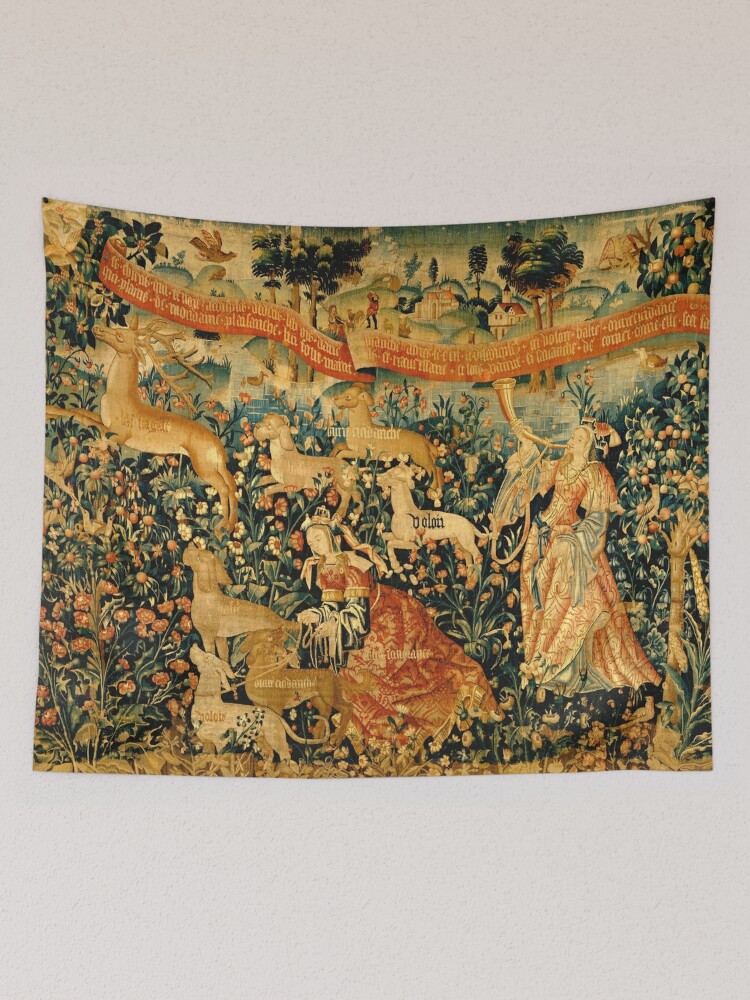The image, a rectangular tapestry taller than it is wide, showcases an intricate forest scene populated with a variety of elements. Set against a grayish tan background, the tapestry prominently features two women dressed in ornate, medieval-style dresses with headpieces. One woman, positioned on the right, is playing a bugle, while the other, in the center, appears seated. Surrounding the women are six dogs, some of which have small, unreadable Latin inscriptions on their bodies. On the left side of the tapestry, near the corner, stands a deer with antlers, seemingly being pursued by one of the women and the dogs. 

A red banner with Latin text decorates the upper portion of the tapestry along with a distant view of a small village, castle-like structures, trees, and birds flying in the sky. The scene is richly detailed with various flowers, fruits, and what resembles wheat adorning the green landscape. The bottom of the tapestry hints at more dogs and possibly a goat, enhancing the medieval pastoral ambiance. The entire composition exudes a sense of nature intertwined with human activity, typical of Middle Ages artwork.